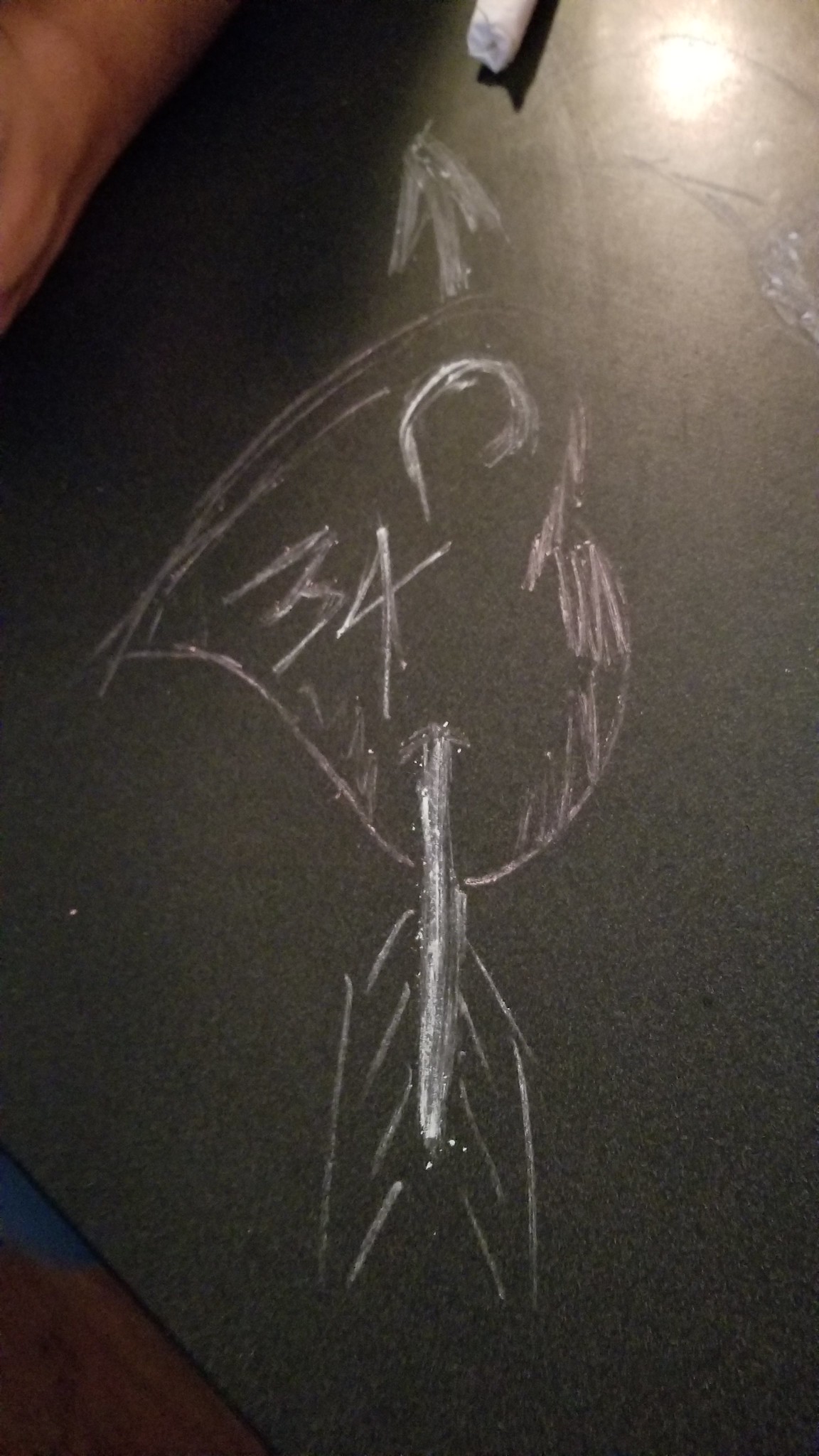A detailed and descriptive caption for the image:

"A chalk drawing on a blackboard, prominently featuring a charming pink heart outlined in bold strokes. Piercing through the heart is a carefully depicted arrow with a traditional arrowhead at its tip and two triangular feathers at the back. Above the drawing, a piece of white chalk rests, hinting at the artist's medium. Within the heart's outline, faint chalk marks suggest a number '3' and intriguingly ambiguous shapes, which could be interpreted as a '4' or as the symbols 'X' and 'D'. The overall composition conveys a whimsical, love-struck illustration, evoking traditional romantic imagery."